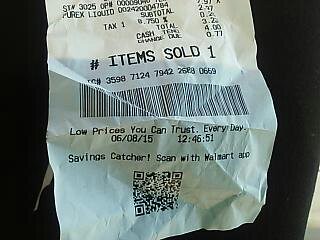This is a detailed close-up photograph of a crumpled receipt printed on thermal paper, issued by Walmart. The receipt is noticeably wrinkled and has multiple creases, lying against a dark, solid background. Key details visible on the receipt include the purchase of "Purex Liquid," with a subtotal amount listed as $2.00 and the tax calculated at 7.50%, amounting to a total of roughly $3.20. The cash tendered is shown as $4.00, and the change due is mistakenly printed as $77.00, which appears to be an error. One item was sold at a price of $1.00. Below this information is a long string of numbers followed by a barcode. Beneath the barcode, the text reads "Low prices you can trust every day." The date on the receipt is June 8, 2015, and the time is stamped as 12:46:51. There is also a note prompting users to use the "Savings Catcher" feature by scanning the receipt with the Walmart app.